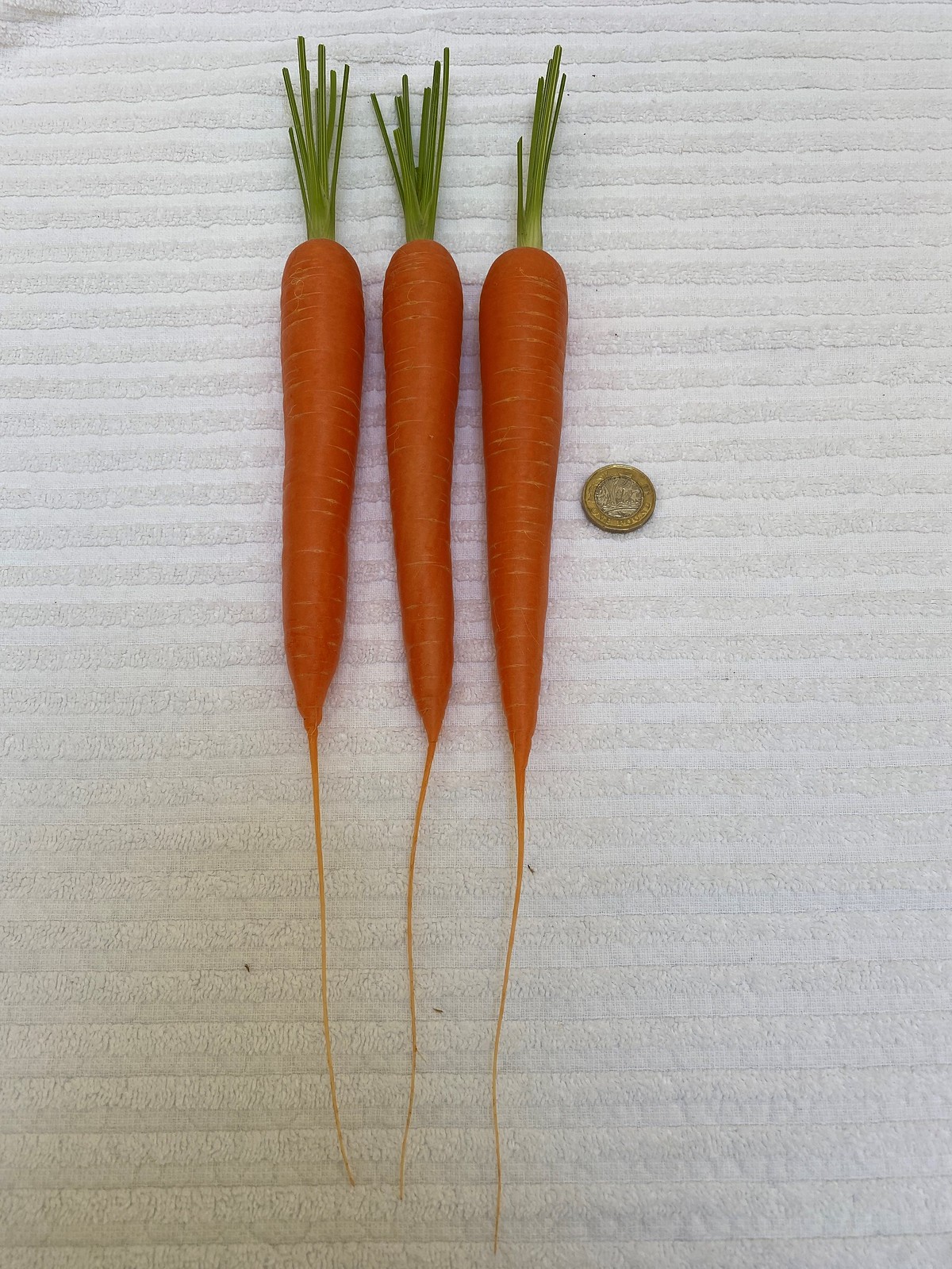The image features three meticulously arranged, vibrant orange carrots with their green stems intact, laid out horizontally in a neat row on a textured white cloth. Each carrot exhibits a uniform size, approximately six to seven inches in length, characterized by long, trailing stringy roots extending from their tips. The green tops are neatly trimmed, extending about three inches above the carrot bodies, with each stem branching out into multiple segments. Positioned to the right of the carrots is a bimetallic coin with a gold edge and a silver center, akin to the older one-pound sterling coins used in Great Britain. This coin, with engraved text along its edge and a sculpted head in its center, provides a size reference, indicating that each carrot is roughly five times the length of the coin. The white cloth beneath displays a subtle striped texture, though it appears slightly yellowed in the bottom left corner, adding to the overall natural and rustic feel of the image.